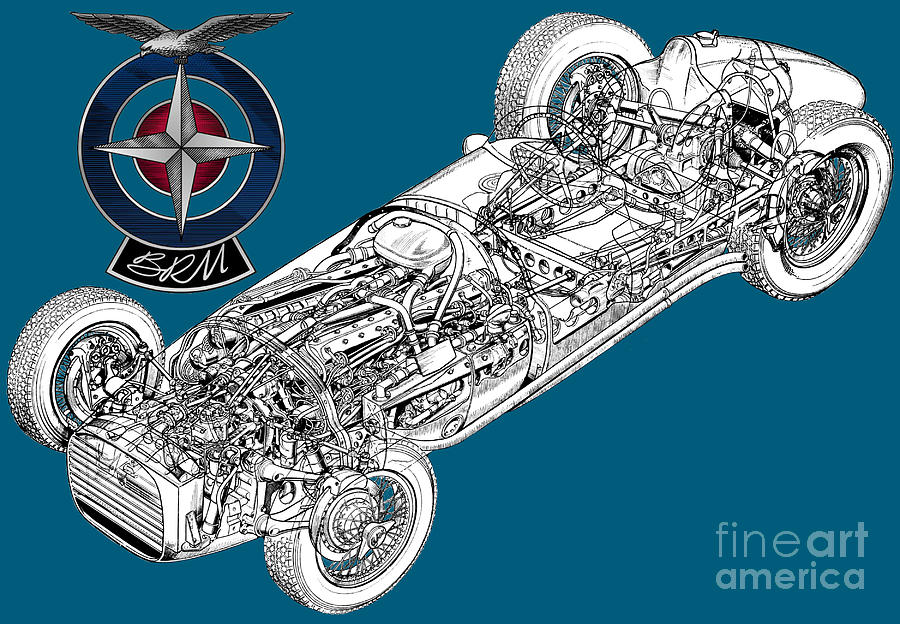This image is a detailed, digitally created color graphic featuring a black and white pencil illustration of the inner workings of a go-kart. It is set against a medium blue background. The go-kart, which is a long, narrow motorized vehicle with four wheels, two in the front and two in the back, is depicted diagonally from the bottom left to the top right. The single seat is positioned between the rear wheels, with a steering column and space for legs towards the front. The majority of the vehicle's structure comprises a long, narrow section housing the engine, showing all the internal parts, wires, and connecting cables, much like a schematic drawing.

In the upper left corner of the image, there is a logo featuring a blue and red circle with a silver four-pointed cross in the middle, topped by a silver eagle with its wings spread. Beneath this logo are the letters "BRM." The words "Fine Art America" are printed in the lower right corner. The colors present in the image include various shades of blue, red, black, white, and silver, and the overall graphic appears to be digitally rendered.